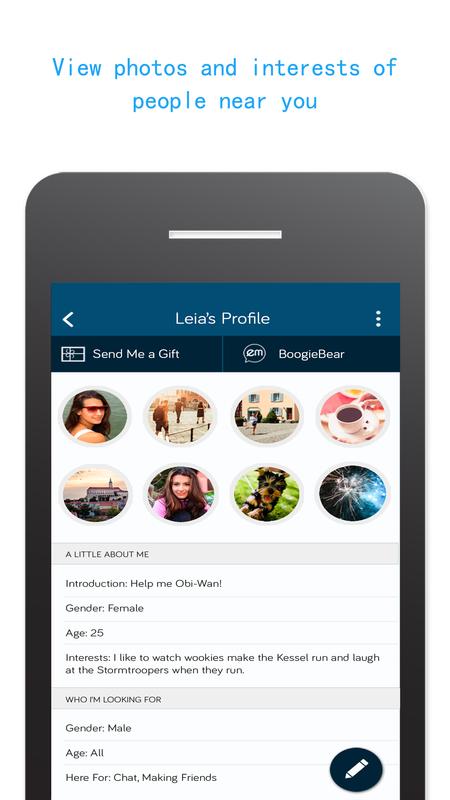Against a white background, at the top center of the image, there is a phrase in fluorescent light blue: "View photos and interests of people near you". Approximately four lines down, a vertical dark gray oval is visible. In the same centered alignment, about four lines from the top, is a short, thick white line. Descending around three lines below that, a dark blue rectangle appears. At the bottom left of this rectangle is a white left-pointing arrow, while the center displays the text "Layla's Profile". To the right, there are three vertical dots indicating an ellipsis. 

Below this section, there's a black banner containing two buttons with icons on the left. The button on the left is labeled "Send Me a Gift" and the one on the right is "Boogie Bear". 

Further down, a light gray rectangle is present. It contains two rows of four profile icons each at its top. Below this, on a gray banner, the text reads "A Little About Me". The introduction section states: "Help me, Obie Dashwani". Below are details listed as "Gender: Female" and "Age: 25". Tiny text beneath provides interests: "I like to watch Wookies make the Kessel Run and laugh at the stormtroopers when they run".

Under this, another gray banner with the text "WHO I'M LOOKING FOR" appears in all caps. It specifies "Gender: Male", "Age: All", and "Here for: Chat, making friends". Situated on the right side of this section is a black circle featuring a white pencil icon inside.